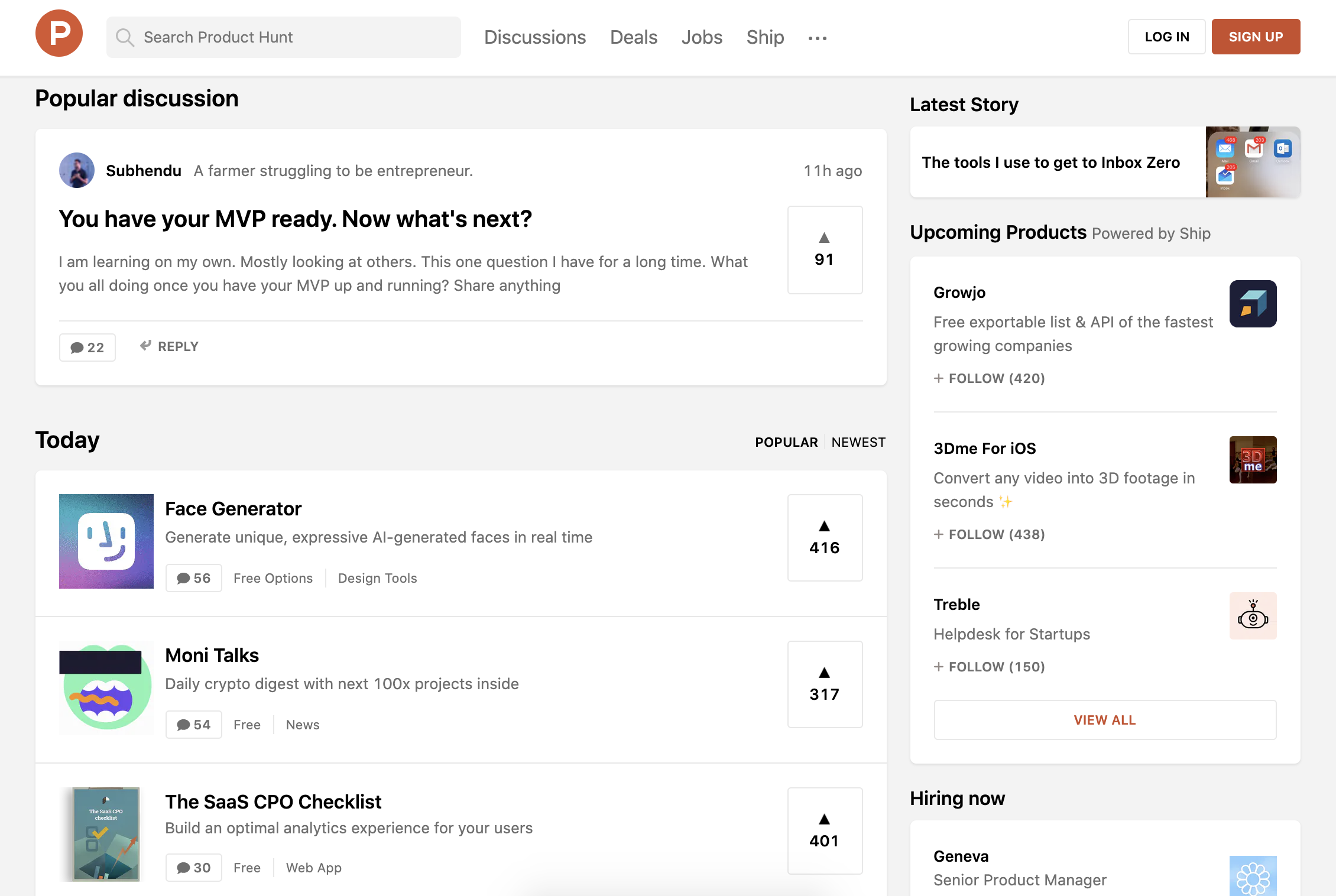A detailed description of the webpage could be structured as follows:

---

Screenshot of a multifaceted online platform combining elements of an app store, social media, and news aggregation. The top navigation bar features tabs labeled "Discussions," "Deals," "Jobs," and "Ship," suggesting a diverse range of services. 

Prominently displayed in the center is a popular discussion thread titled "You have your MVP ready. Now what's next?" with a user seeking advice on next steps after launching their Minimum Viable Product. The post mentions self-learning through observation and asks the community to share their post-MVP strategies.

On the right-hand side, a section titled "Latest Stories" lists articles such as "The tools I used to get to Inbox Zero." Below it, upcoming products like Grojo, 3DME for iOS, and Treble are highlighted.

Further down on the right, there's a "Popular Apps Today" section featuring apps such as Face Generator, 3DTalks, MONITalks, and the SAAS CPO Checklist. 

In the bottom right corner, a "Hiring Now" box advertises a Senior Product Manager position at Geneva, indicating job listings as part of the site's offerings.

Overall, the site appears to serve as a comprehensive resource for app discovery, tech news, community discussions, and job opportunities, catering to tech enthusiasts and professionals alike.